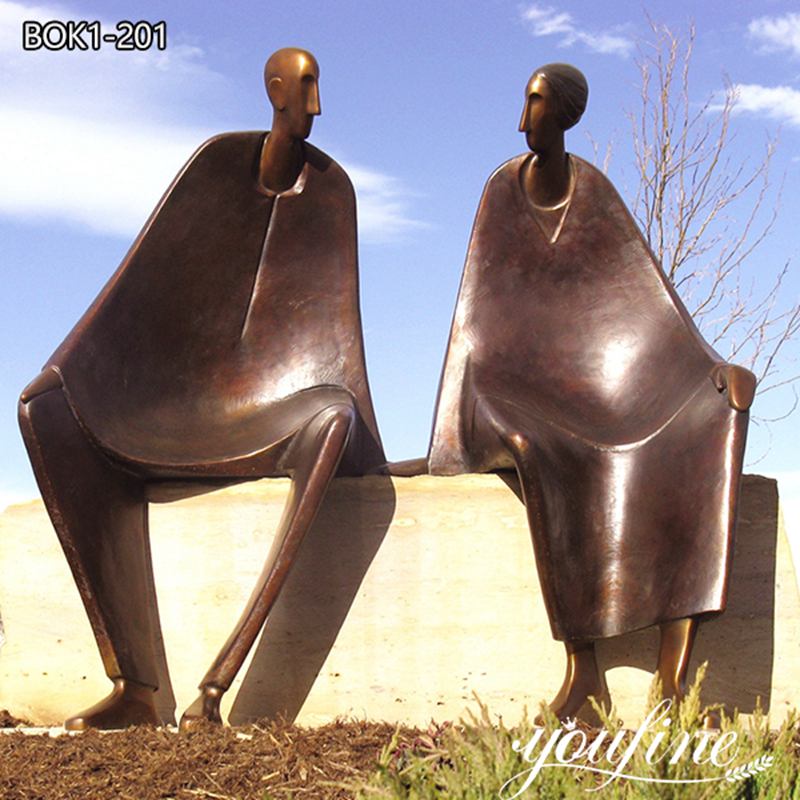In this outdoor photograph, set against a backdrop of a blue sky adorned with white clouds, we see a distinctive scene featuring two bronze or copper statues perched on a large concrete pedestal. These statues, a man and a woman, both with bald heads, elongated necks, and long noses, are depicted in a sitting position, facing each other. The man's figure includes a cape-like drape that falls to his knees, and his thin legs, dressed in pants and shoes, extend down to the ground with one hand resting on his knee and the other on the pedestal. The woman's sculpture, adorned in a dress, similarly extends to the ground but appears to be barefoot. Their chest and stomach areas are concave, creating a bell-shaped torso, and their laps are designed wide enough to potentially serve as makeshift seats, although using them as such is likely impractical due to the heat from the sun. The foreground of the picture shows a grassy area interspersed with mulch and dirt, while a thin, leafless tree with wispy branches can be seen nearby, contributing to the serene and artful ambiance of the setting.